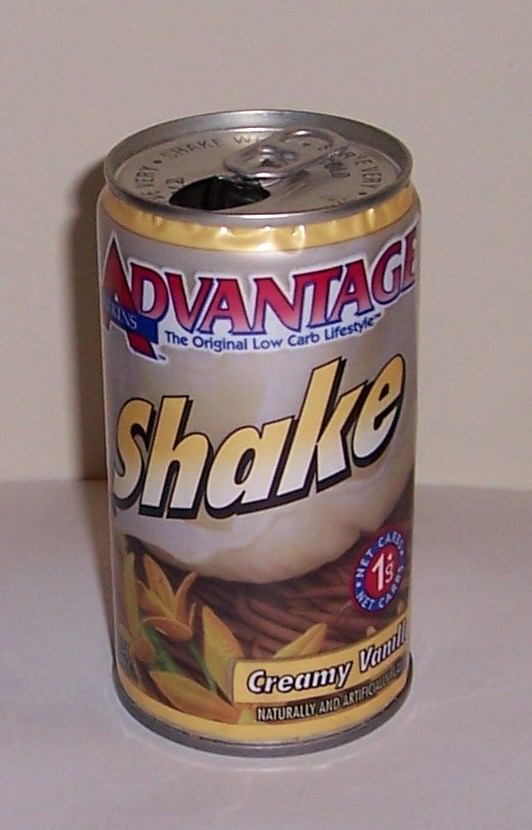This image features an opened can prominently displayed on a counter. The counter and the wall in the background share a similar off-white, creamy hue, providing a neutral backdrop. The can, labeled "Advantage Atkins" and promoting "The Original Low Carb Lifestyle," serves as the focal point. The word "shake" appears midway on the can, starting in a yellow gradient that transitions to white. At the bottom of the can, the flavor is identified as "Creamy Vanilla," both naturally and artificially flavored. A small circular label on the side highlights "Net Carbs: 1 Gram." Additionally, near the base of the can, there are illustrations of flowers, likely vanilla bean flowers, adding a decorative element.